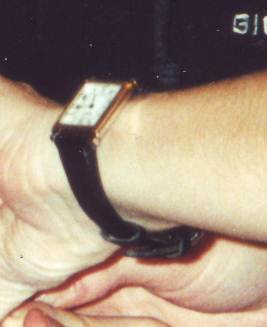Three hands stacked on top of one another, symbolizing unity and support. The bottom hand has visible wrinkles, showcasing age and experience. The middle hand sports a bronze watch with a white clock face; the hour hand points to the left and the minute hand is angled upwards to the left. The watch has a black strap fastened securely through loops. The topmost hand rests gently, completing the trio of connections.